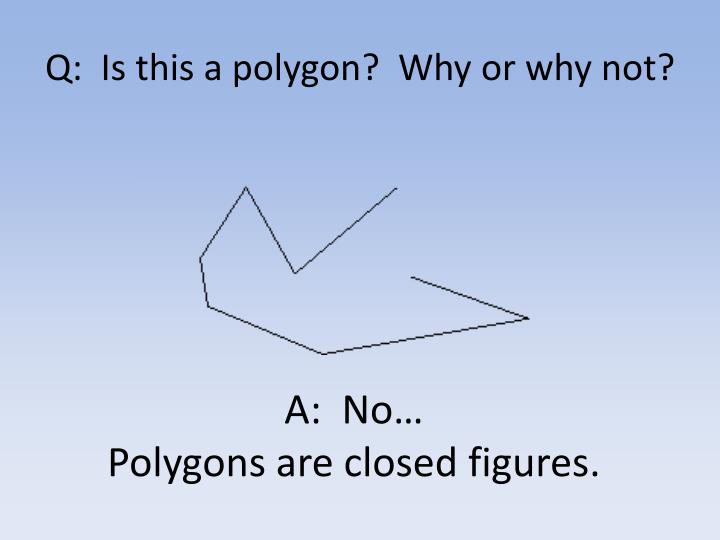The image features a bluish fading into gray background, overlaid with black text and a geometric shape. The top of the image displays black lettering formatted as "Q: Is this a polygon? Why or why not?". Centered in the middle is a shape composed of eight sharp-angled lines that do not connect, forming an open figure. The bottom section of the image contains the text "A: No... Polygons are closed figures." The overall layout resembles a test question from a textbook, asking if the depicted shape qualifies as a polygon, with the explanation that it does not because it is not a closed figure. The design is simple, with no border or additional images, focusing solely on the question and the open geometric shape against the gradient background.